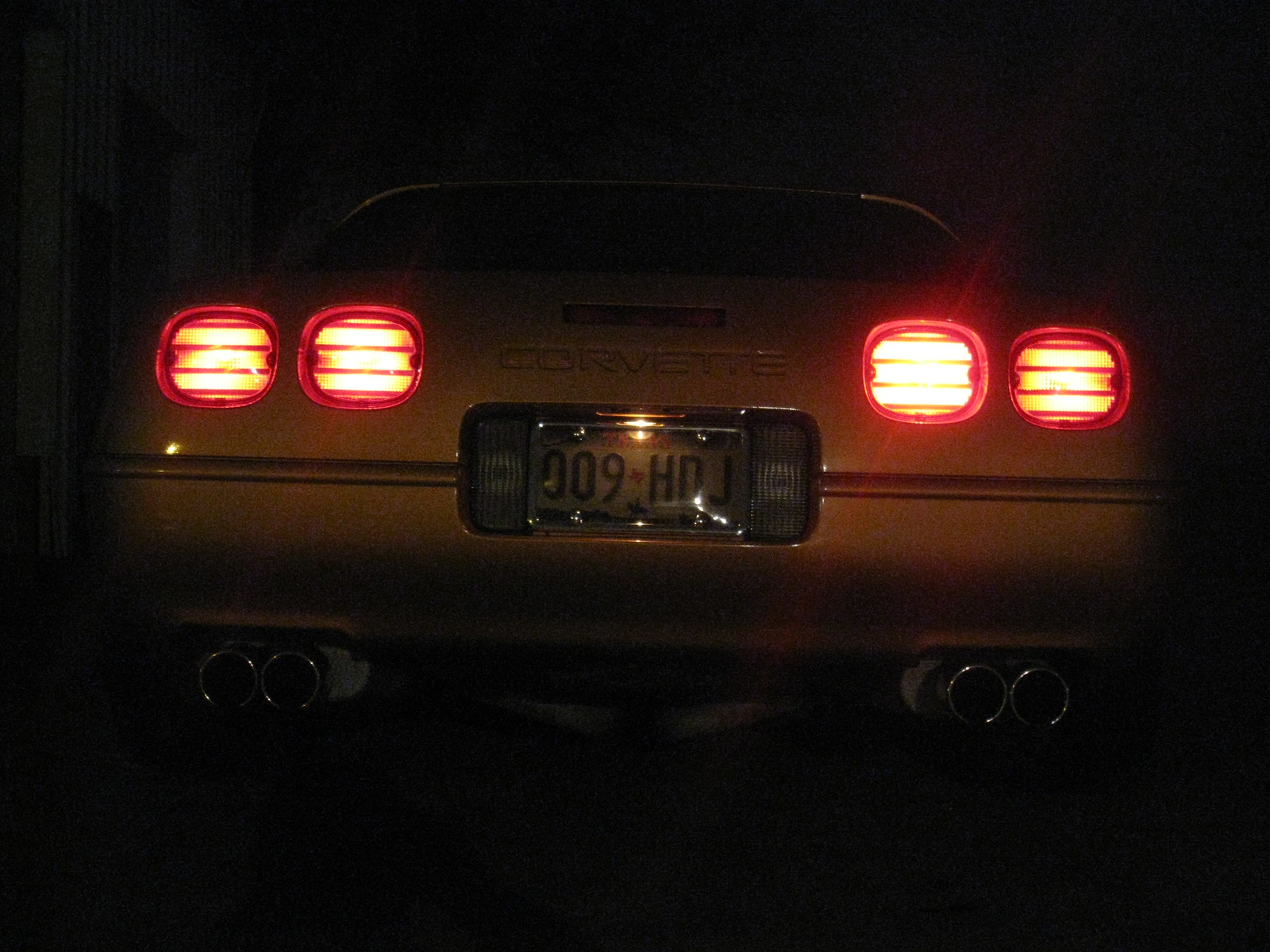The photograph depicts the rear of a Corvette, captured in a dark setting, either at night or in a dim parking garage. The car appears to be likely white or possibly a light color, although the low lighting makes it difficult to ascertain definitively. The prominent "Corvette" emblem is embossed above a license plate that reads 009 HDJ, with a small red emblem suggesting the state of Texas between the characters. The illuminated rear consists of four lights arranged symmetrically: two on the left and two on the right of the "Corvette" text, each featuring a reddish circular shape with yellow bands, and resembling rounded rectangles. Beneath these lights and the license plate, there are two pairs of shiny exhaust cylinders, adding to the classic look of the vehicle.